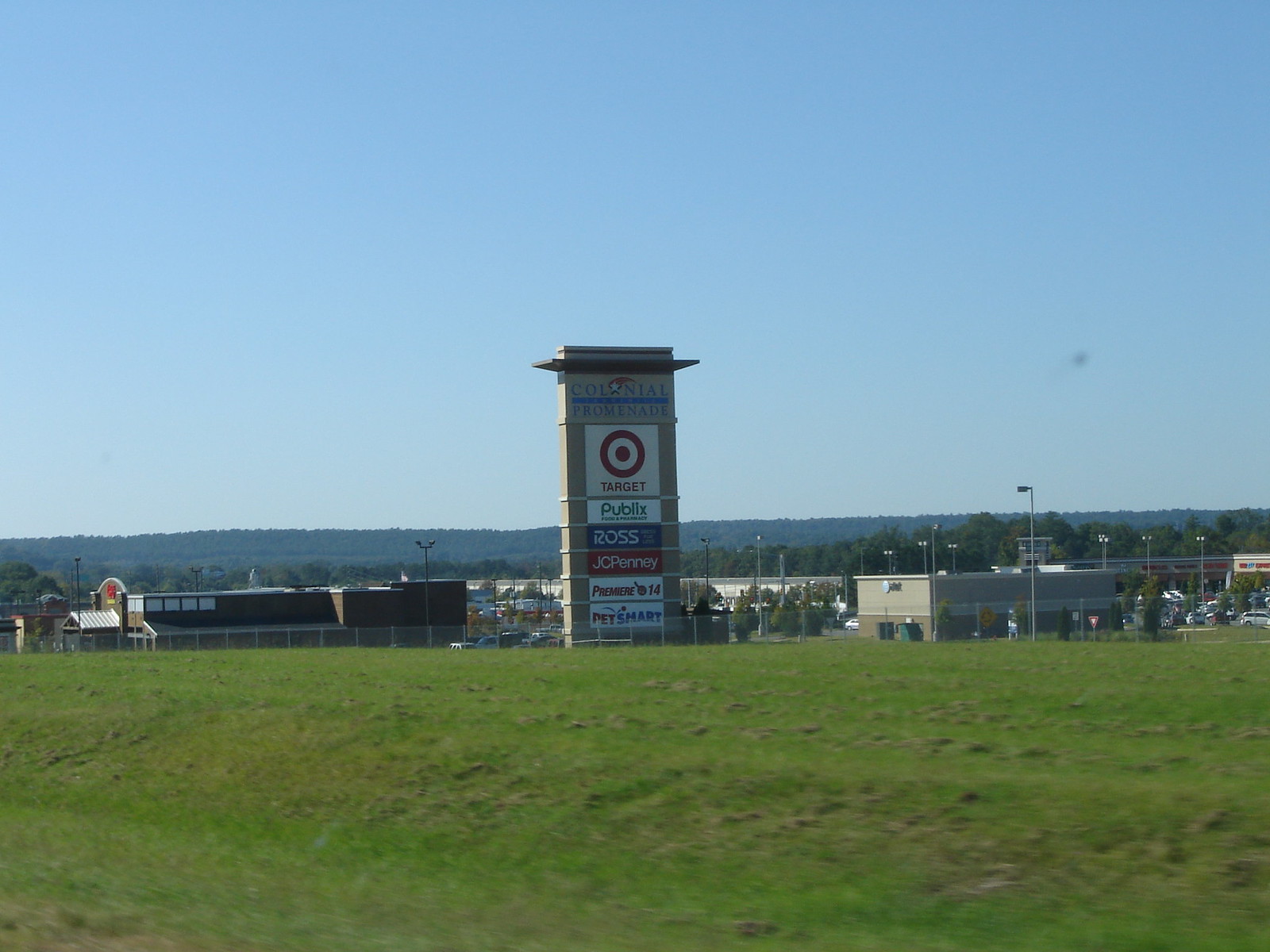The image showcases a bustling shopping center, prominently featuring a large, contemporary sign visible from the highway. This sign, likely photographed by a passerby, appears to read "Colonial Promenade." The sign vividly lists several stores, starting with Target emblazoned in a bold, square logo. Below, the familiar green and white of Publix is followed by the fashion retailer Ross. JC Penney’s logo stands out with its red background and white text. Although one store name is unreadable, PetSmart, with its red and blue text on a white background, is prominently displayed. The shopping center itself, distant but visible beyond the sign, is nestled amidst some trees, offering a glimpse of its sprawling layout.